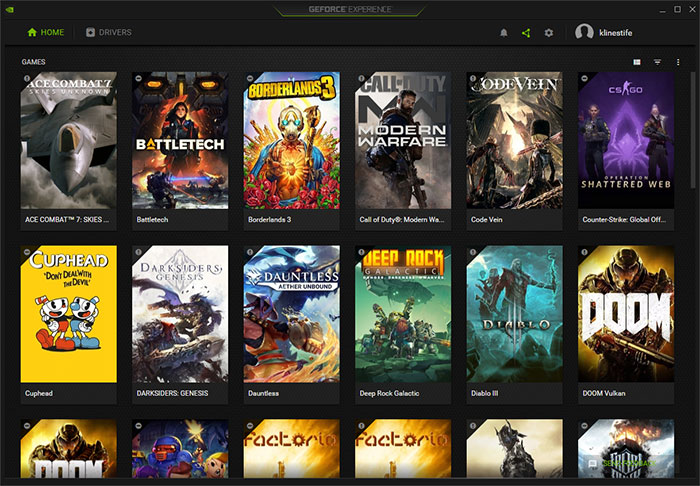The image appears to be a screenshot from a gaming platform, possibly NVIDIA GeForce Experience, as indicated by the prominent logo at the top. The user interface includes several icons: a green home icon, a non-highlighted Drivers section, notifications bell, a green Share button, a settings cogwheel, and a profile picture with the user's name.

The main content showcases a library of games arranged in three rows, each containing six titles. However, the third row is only partially visible, cutting off some game names. The visible games include:

1. ACE COMBAT
2. BATTLETECH
3. BORDERLANDS 3
4. CALL OF DUTY: MODERN WARFARE
5. BATMAN: ARKHAM KNIGHT
6. COUNTER-STRIKE: GLOBAL OFFENSIVE - SHATTERED WEB
7. CUPHEAD: DON'T DEAL WITH THE DEVIL
8. DARKSIDERS GENESIS
9. DAUNTLESS
10. DEEP ROCK GALACTIC
11. DIABLO III
12. DOOM

These games predominantly feature action-packed, combat-oriented themes, with characters often adorned in battle gear. The overall tone is intense and dark, with the exception of "Cuphead: Don't Deal with the Devil," which, despite its potentially sinister title, is presented with a charming and whimsical art style.

This detailed layout of the user interface and game selection highlights the platform's emphasis on high-octane, immersive gaming experiences.